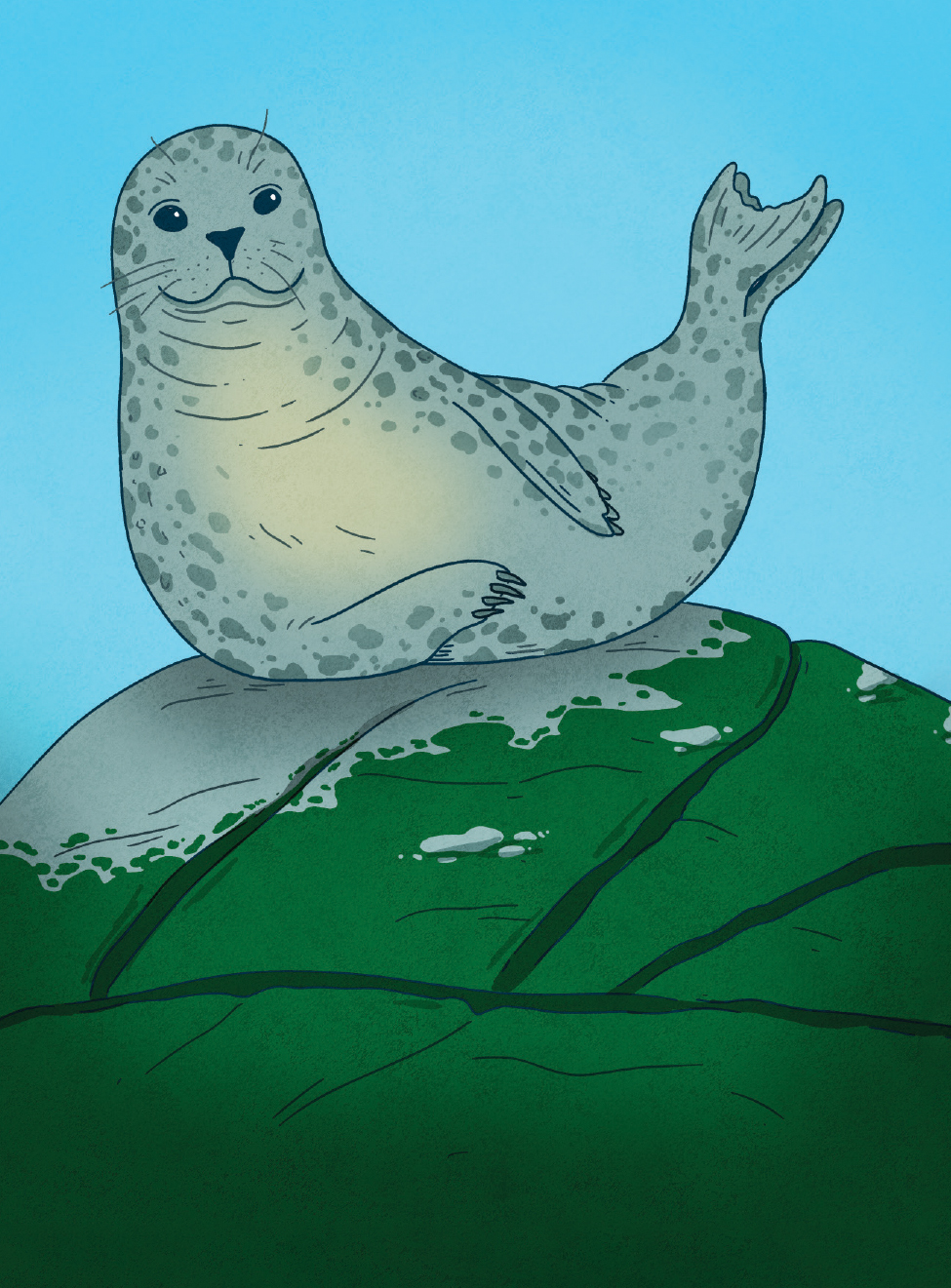This image is a detailed digital rendering of a smiling seal sunbathing on a rock. The seal, drawn with a cartoon-like style, is depicted laying on its side with its tail in the air and large expressive black eyes. It has a mottled gray body with a light tan belly below its neck and a distinctive black triangular nose. The rock, which occupies the bottom half of the image, is predominantly green with patches of gray, suggesting the presence of algae. The background is a clear, light blue sky, adding contrast to the vividly colored seal and rock. The overall scene is vibrant and detailed, showcasing the seal resting happily on its perch, lending a cheerful and peaceful mood to the composition.